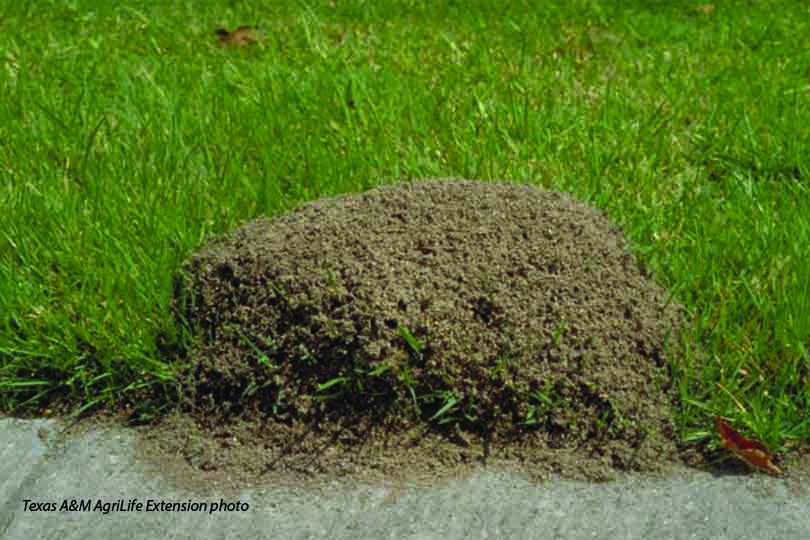The photograph captures a well-maintained, lush green yard, featuring what appears to be Bermuda grass. Along the edge of the yard is a gray, textured sidewalk. Dominating the center of the image is a large, prominent fire ant mound, measuring approximately 12 inches in length and 5 to 7 inches in height. The mound, which is brown with various protrusions, extends from the grass and partially covers the sidewalk. Scattered around the grass are a few leaves. Notably, the bottom left corner of the image includes an italicized credit in black font, reading "Texas A&M AgriLife Extension Photo." The photograph is taken during the daytime and does not show any visible ants.